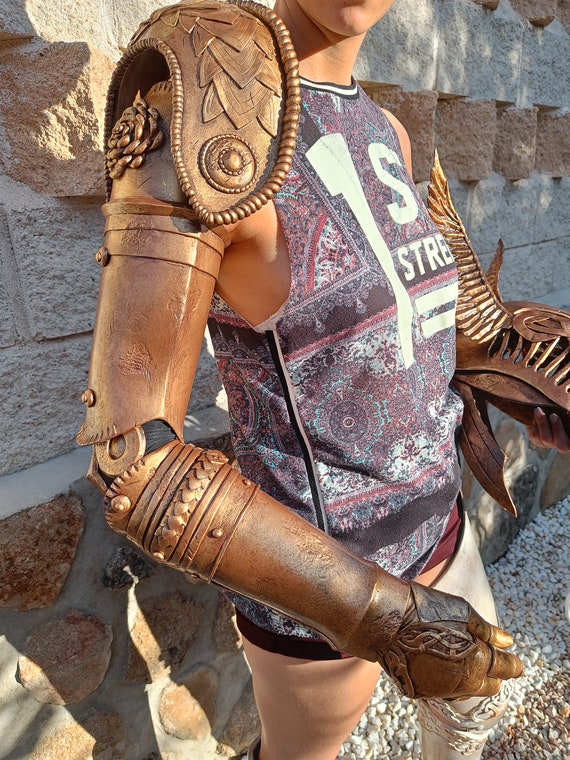This image is a close-up shot of a very thin woman with light skin standing against a concrete block wall, wearing a costume that resembles a metal gladiator suit. The photograph captures her from just below her chin to slightly above her knees. She is adorned in a blue tank top with pink accents that boldly displays the words "First Street" across her chest. Her attire includes very short shorts, revealing a portion of her white thigh. 

On her right arm, she wears an elaborate gold-colored gladiator sleeve that extends from her shoulder down to her hand. The sleeve features intricate, ornate designs and bends at the elbow, with a prominent shoulder piece adorned with a rose. She holds a gladiator helmet in her right hand, which has golden wing-like earpieces.

Her left leg appears wrapped in a protective white material that resembles a cast, while her right leg remains uncovered. The woman’s costume boasts textured, metallic-looking designs that give an impression of both leather and metal, contributing to her striking, mythic appearance.